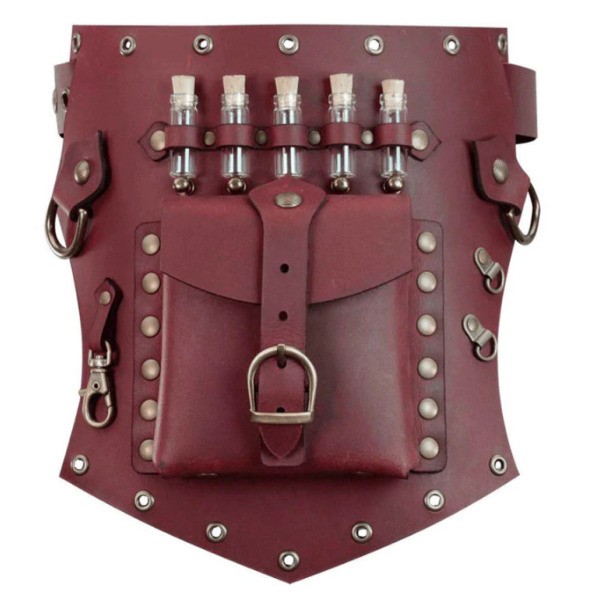The image features a deep red burgundy leather pouch designed to be worn on a belt. It is intricately detailed with numerous metal elements, including brass brads, circular grommets, and D-rings. The pouch is adorned with 7 grommets along the top and bottom edges. The main compartment is secured with brass brads and can be unbuckled to store small items. On the upper half of the pouch, there are 5 cylindrical glass vials, each corked and securely held in place by the leather. The sides feature various hooks and keychain latches, providing multiple points for attachment. The bottom of the pouch tapers to a point, giving it a sleek and functional design ideal for carrying small, essential items.